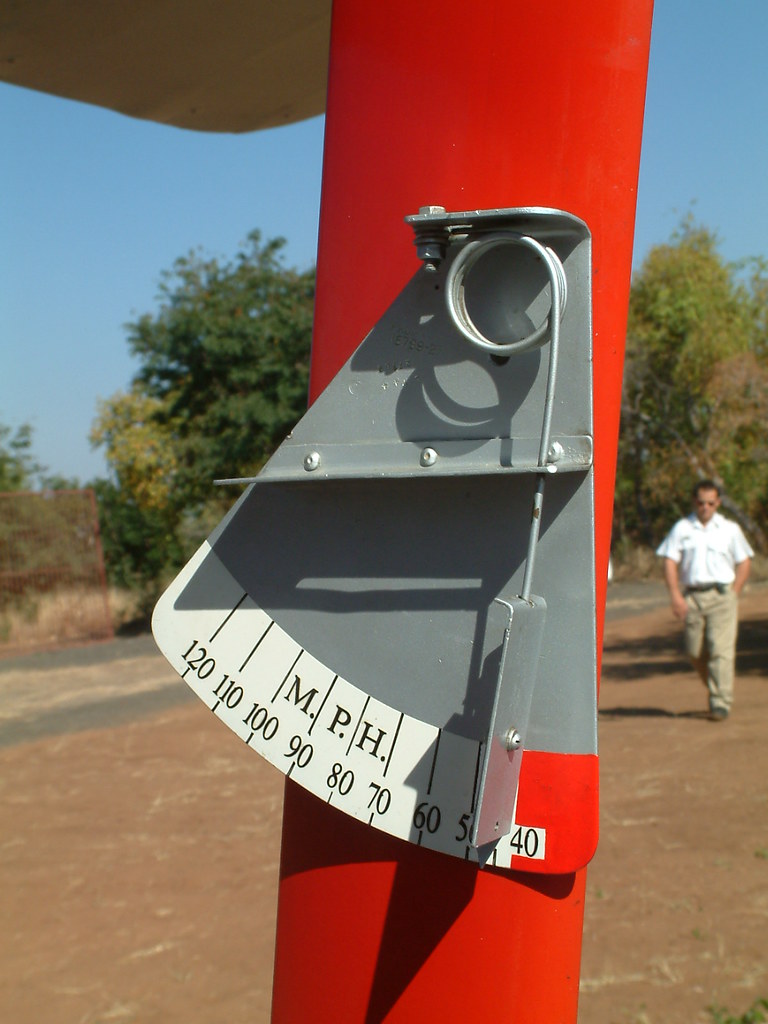A vibrant outdoor scene captures a clear blue sky accented by large, lush trees in the background. A street with a concrete divider runs through the middle of the image, bordered by a concrete walkway. On this walkway, a man is strolling while wearing khaki-colored pants and a white, short-sleeved shirt. He sports glasses and has short dark hair. Prominently featured in the foreground is a large red pole with a triangular silver attachment on its side, from which a metal cord extends downward. This setup includes a white background with black writing and labels indicating speeds from 120 miles per hour down to 40, highlighted with red markings at the lower end. The adjustable indicator seems to measure the speed of pedestrians. The man is approaching this intriguing post, which has a light brown component extending from its base.